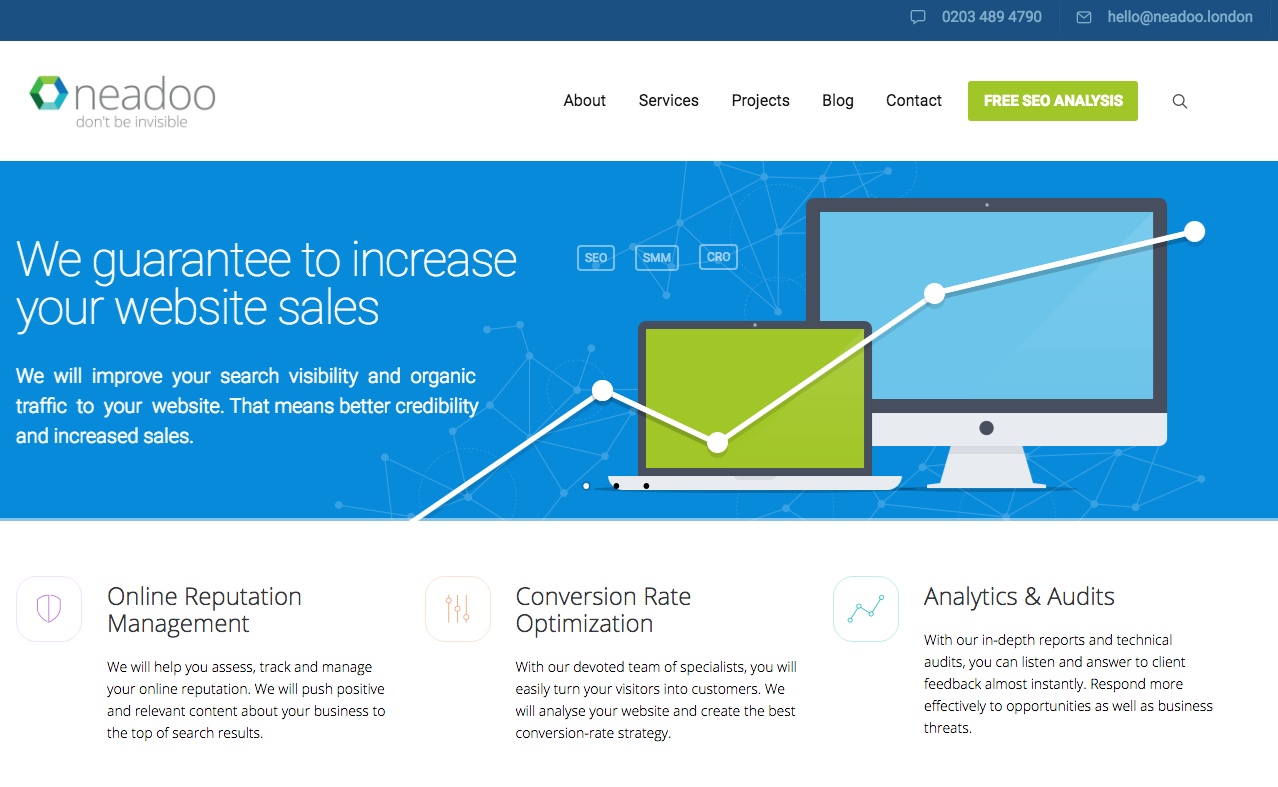This is a detailed description of a website's homepage:

The top of the website features a prominent blue banner stretching across the width. On the left-hand side of this banner, there's a contact phone number accompanied by an email address, "hello@neadoo.london." Below the main banner, also on the left-hand side, is the company's logo, "neadoo," in lowercase letters, followed by their tagline, "don't be invisible."

Directly beneath the blue banner is a white navigation bar containing links labeled "About," "Services," "Projects," "Blog," and "Contact." Positioned towards the center-left of this bar, there's a green button with white text that reads "Free SEO Analysis," alongside a magnifying glass icon.

Dominating the center of the homepage is a large blue section. On the right side of this section, there are images of a desktop computer with a blue background screen and a laptop with a green background screen. On the left side of this blue section, there is prominent white text stating, "We guarantee to increase your website sales. We will improve your search visibility and organic traffic to your website. That means better credibility and increased sales."

At the bottom, three service categories are listed, each with an accompanying icon and a brief description:
1. **Online Reputation Management** 
2. **Conversion Rate Optimization**
3. **Analytics and Audits**

Each category includes a paragraph providing more detailed information about the respective service.